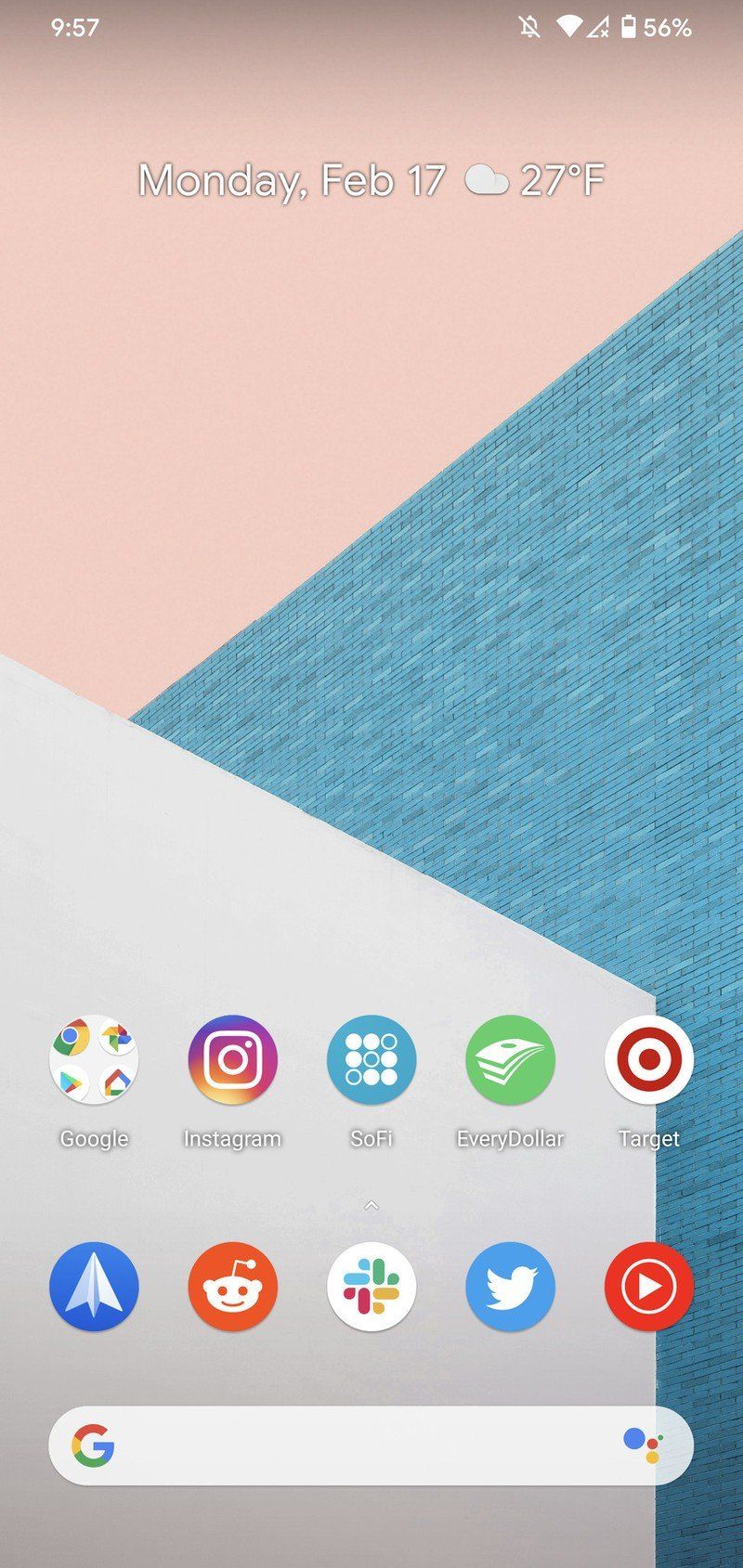A mobile screenshot captured at either 9:57 a.m. or p.m. showcases a diverse and aesthetically pleasing background featuring geometric shapes, reminiscent of a sunrise sky with hues of pink and blue. The interface indicates various icons including Google, Instagram, SoFi, EveryDollar, Target, Reddit, Twitter (or X), YouTube, and Telegram, displayed in a row. At the top of the screen, notification symbols for a silenced phone, Wi-Fi connection, and a battery level of 56% are visible, along with the date, Monday, February 17th, and the temperature, a chilly 27 degrees Fahrenheit with cloud cover. The white text contrasts well against the pinkish background, making it easy to read. Beneath the row of app icons, a Google search bar resides. No additional text is present on the screen.